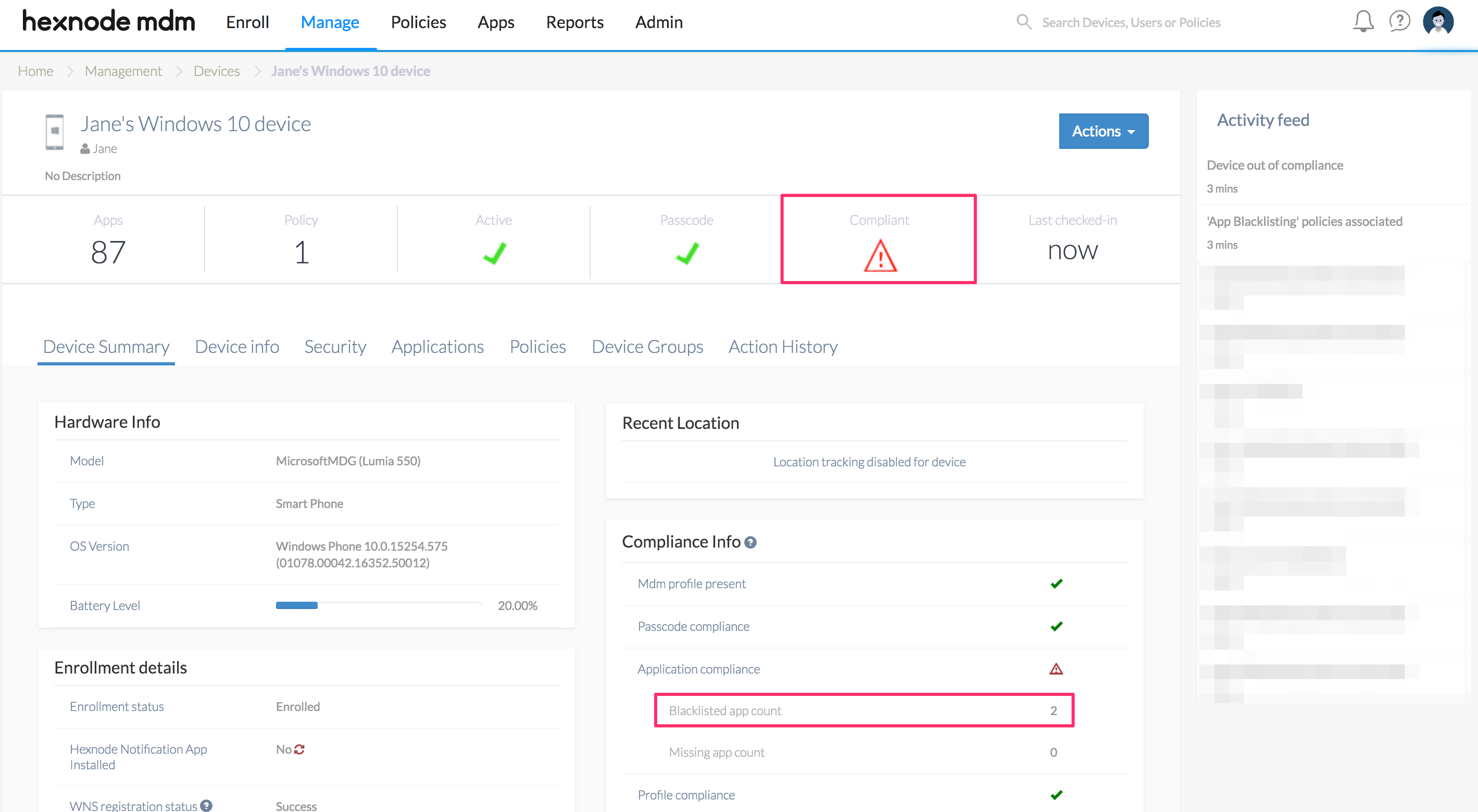Details about Jane's Windows 10 Device are displayed on the screen. 

At the top left, "Hexnode MDM Enroll" is prominently displayed, with blue text heading categories like "Manage," "Policies," "Apps," "Reports," "Admin," and "Mental Health." Below, main sections include "Search Devices," "User Policies," "Home," "Management Devices," and "Jane's Windows 10 Device."

In the detailed view, Jane's device is identified as a "Smartphone." The dashboard lists "87 Apps," "Policy 1" which is marked as "Active" with an open checkmark, and "Passcode" also indicated with an open checkmark. A red square symbolizes a "Complaint." 

The navigation panel provides comprehensive device information: "Device Summary," "Device Info," "Security," "Applications," "Policies," "Device Groups," and "Action History." 

Highlighted hardware details specify it as a "Fixed Model: Microsoft MDG, Lumia 550" with the type being "Smartphone" and the OS version as "Windows Phone 10." The battery level is noted at "20%," and enrollment details confirm "Enroll Text on Amazon" as "No." 

Moreover, "Device Restriction Success Compliance Info" is displayed. The status of "MDM Profile" is marked as "Permanent Check," and "Passcode Compliance Check" is indicated alongside "Compliance Info." 

There's mention of two apps under compliance: "Blacklisted App Account: 2" and "Missing App Account: 0," followed by "Profile Compliance" with a green checkmark. It's also noted that "Location Checking" is disabled for the device.